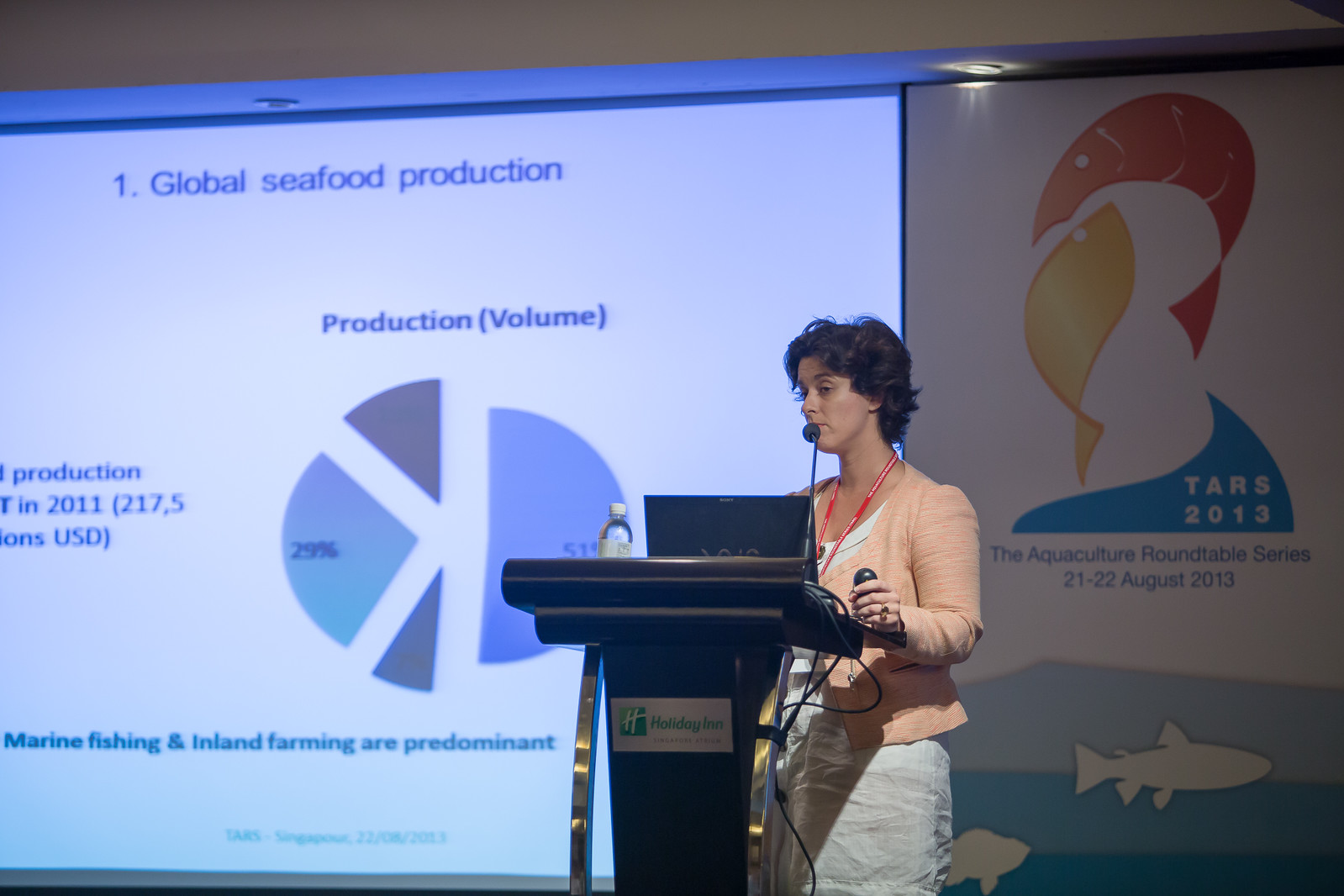In this detailed photograph, a woman is seen delivering a presentation indoors. She stands at a podium, speaking into a headpiece microphone, and appears to be holding a clicker in her hand. The woman is dressed in a light orange jacket over a white shirt, paired with a white skirt. On the podium, there is a plastic bottle of water and a laptop.

Behind her, a large screen dominates the background, displaying a comprehensive slide. The slide's header, written in blue, reads "Number One Global Seafood Production." Below it, there is a pie chart predominantly in shades of blue, depicting production volumes with categories such as marine fishing and inland farming. The chart mentions data from 2011, citing a production volume of 217.5 US units, though some parts of the text are not clearly legible. 

To the right side of the screen, a logo features two fish in shades of orange and yellow, accompanied by the text "TARS 2013." Below the logo, it reads "The Aquaculture Roundtable Series - 22 August 2013," with a small wave design and two smaller white fish illustrations beneath it.